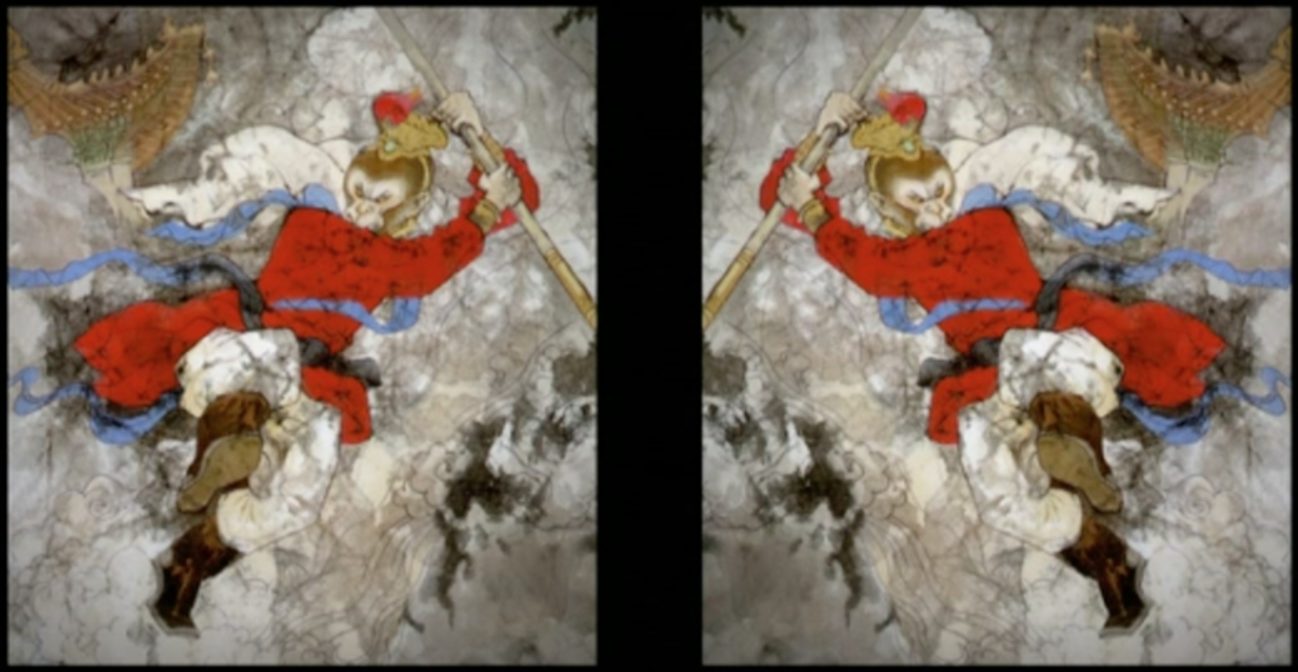The image is a richly colored fantasy painting, rectangular in shape with its longest side horizontal. Dominating the composition is a central, wide, vertical black line that bisects the canvas, creating a mirror image of a demon-like monkey warrior adorned in identical attire on both sides. The warrior is dressed in a striking red jacket, white pants, and brown boots, while carrying a staff that seems to mimic bamboo. Each mirrored figure holds the staff above, with one extending it to the upper right quadrant and the other to the upper left quadrant. The monkey warrior's head is topped with a distinctive brown and gray hat or crown, adding to its regal and foreboding presence. Encircling the monkey is a swirling backdrop of smoke or clouds, enhancing the mystical atmosphere of the scene. Behind this ethereal fog, one can discern a bridge and what appears to be a wooden ship, further embedding the image in a fantastical setting.